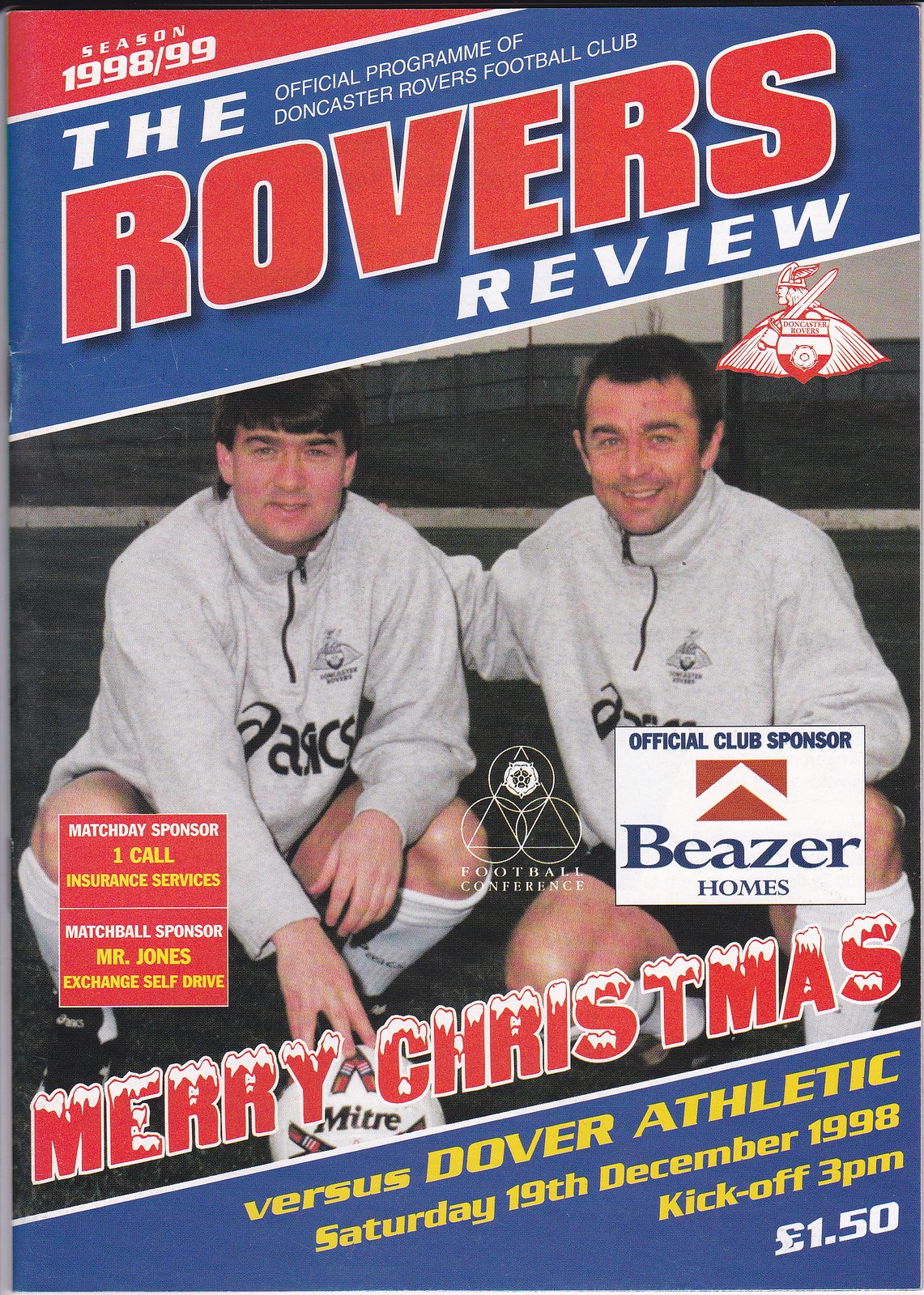The image is the cover of the official program for the Doncaster Rovers Football Club's 1998-99 season, titled "The Rovers Review." The design prominently features red, white, and blue colors. The top left corner clearly states "Season 1998/99." Central to the cover are two men, presumably players, wearing gray three-quarter zip-up sweatshirts with collars, smiling at the camera. The text "Merry Christmas" is displayed festively above the matchup details against Dover Athletic, set for Saturday, 19th December 1998, with a kickoff time of 3 p.m. and a price of £1.50. Additional information includes the official club sponsor, Beaser Homes, match day sponsor, OneCall Insurance Services, and match ball sponsor, Mr. Jones Exchange Self-Drive. The Football Conference logo appears near these sponsors, depicted as three circles with a triangle in the middle.